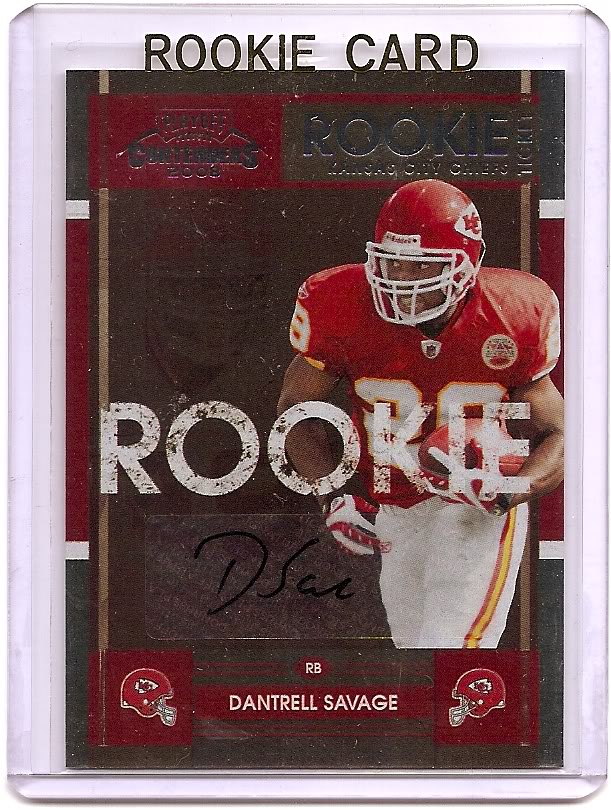The image depicts a rookie football card encased in a clear, protective acrylic sleeve. Dominating the top of the card, against a reflective gold background, are the words "ROOKIE CARD" in black letters. Below this, in the center, the word "ROOKIE" is emblazoned in large, white letters with brown splotches. The card features Downtrail Savage, a player for the Kansas City Chiefs, shown right of center holding a football in his left hand. He is dressed in a full uniform comprising of a red and white jersey and white pants with red and yellow stripes. His signature is located to the left of his legs. At the bottom, Savage's name is displayed in white text, flanked by two team helmets. Additional text lines at the top mention "Player Champions 2008" and "Rookie Kansas City Chiefs." The card's overall color scheme includes dominant shades of red, white, yellow, and gold.